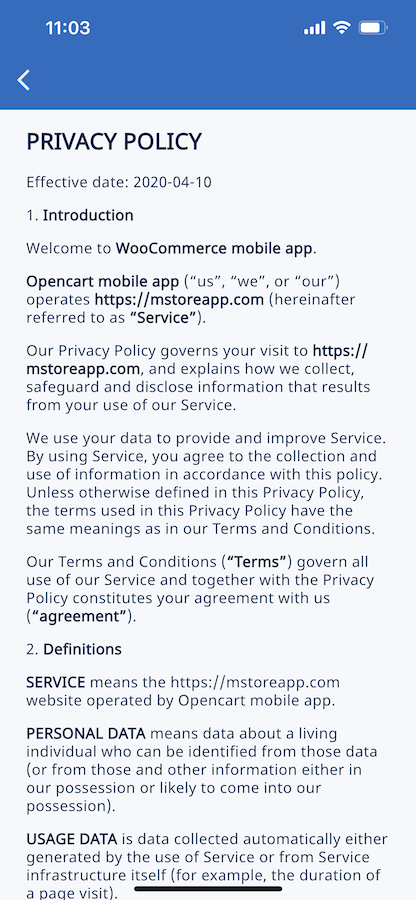This image is a screenshot of an official document titled "Privacy Policy," captured from a mobile device. At the top left corner, the time is displayed as 11:03, while the top right corner shows the cell phone's signal strength and battery life. 

The main body of the document mentions that the effective date of the policy is April 10, 2020. The introduction reads, "Welcome to WooCommerce Mobile App, Open Cart Mobile App, Operates at mstoreapp.com." The policy further explains that it governs visits to mstoreapp.com and outlines how personal information is collected, safeguarded, and disclosed as a result of using the service. The document seems to list various terms related to service agreements, personal data, and usage data.

The background color of the document is white, with all text written in black.